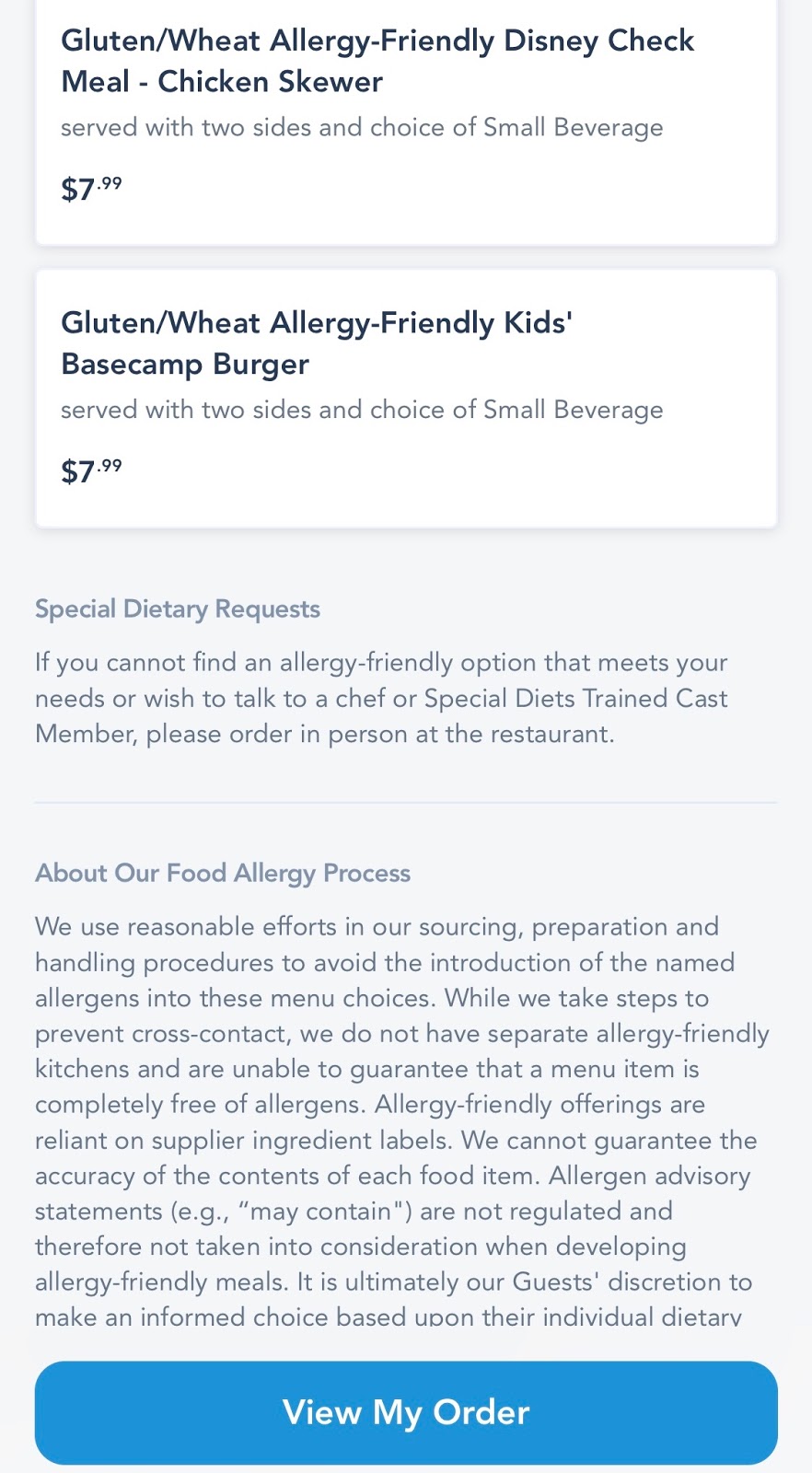On this page, a detailed menu caters to guests with gluten and wheat allergies at a Disney establishment. At the top, the headline reads, "Gluten/Wheat Allergy-Friendly Disney Check Meal." Below this, two meal options are listed:

1. **Chicken Skewer**: Served with two sides and a choice of a small beverage, priced at $7.99.
2. **Kids' Base Camp Burger**: Also served with two sides and a choice of a small beverage, priced at $7.99.

Following the menu items, there is a description addressing special dietary requests. It advises guests who cannot find a suitable allergy-friendly option or who wish to speak with a chef or special diets-trained cast member to place their order in person at the restaurant.

An additional description discusses the food allergy process. It explains that while the establishment uses reasonable efforts in sourcing, preparation, and handling to avoid introducing allergens into the menu items, they do not have separate allergy-friendly kitchens and cannot guarantee that a menu item is completely free of allergens. The allergy-friendly offerings depend on supplier ingredient labels and the accuracy of food content cannot be guaranteed. Guests are ultimately responsible for making an informed choice based on their individual dietary needs.

At the bottom of the page, there is a blue button labeled "View My Order," suggesting that guests review these descriptions before proceeding with their order.